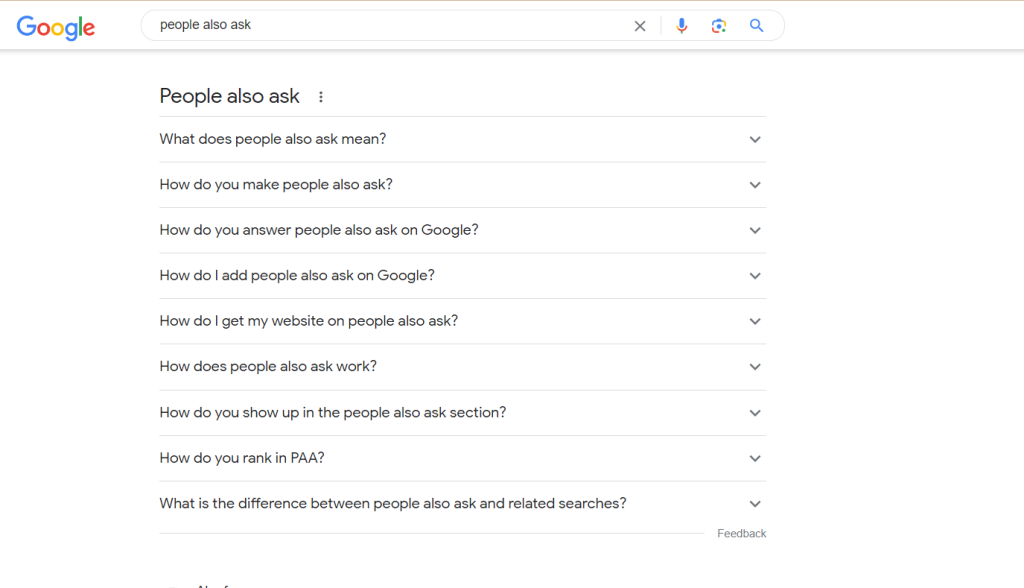The image depicts a Google search results page set against a clean, white background. Dominating the upper left corner is the iconic "Google" logo, rendered in its characteristic vibrant colors. Just to the right, a prominent search bar is displayed, currently showing the query "People also ask." Next to the search bar on the right, a series of icons are arranged: a bright blue and red microphone icon, a secondary icon whose function isn't immediately clear, and a classic magnifying glass search icon.

Below the search bar, there is a vertical list of related queries presented in black or dark gray text. The top line reads "People also ask," followed by a series of specific questions that elaborate on this main query. These include: 
1. "What does people also ask mean?"
2. "How do you make people also ask?"
3. "How do you answer people also ask on Google?"
4. "How do I add people also ask on Google?"
5. "How do I get my website on people also ask?"
6. "How does people also ask work?"
7. "How do you show up in the people also ask section?"
8. "How do you rank in PAA?"
9. "What is the difference between people also ask and related searches?"

In the bottom right corner, there is a "Feedback" link in light gray text, inviting user input on the search results.